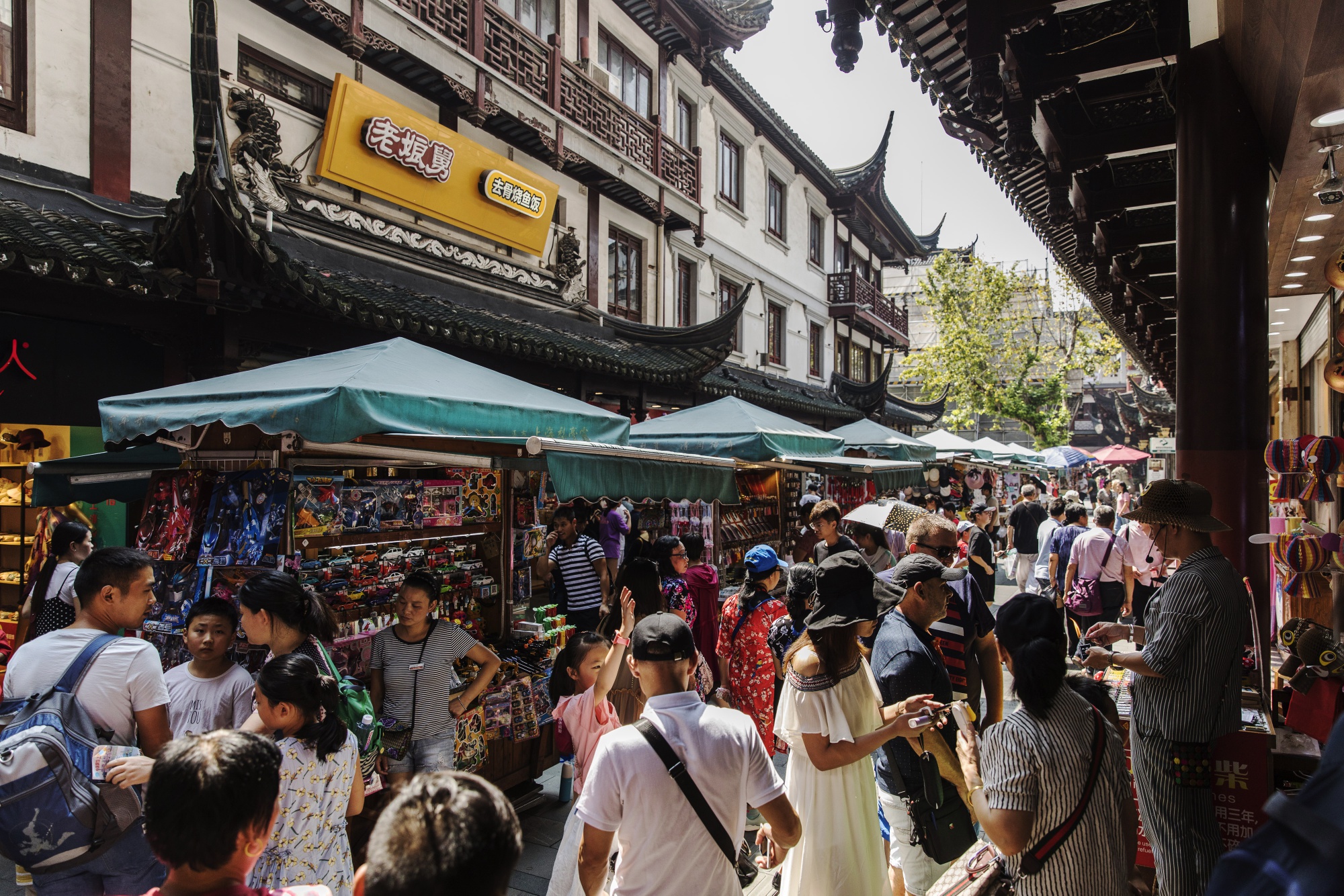This is a color photograph of a bustling street market, likely situated in a Chinese or East Asian city, possibly Chinatown in a Western country. The scene is vibrant and crowded, capturing numerous people engaged in activities such as buying and selling. Many of the individuals appear to be East Asian, with a few Caucasian tourists visible, all dressed in summer attire as the sun shines down brightly. 

The market is set between two buildings; the building on the left has a second story with a yellow sign displaying Chinese characters. The architecture is traditionally Chinese, featuring roofs with curved edges, white walls, and reddish-brown wooden balconies and decorative framing.

Beneath the buildings, green square canopies and turquoise tops cover the countless stalls lining the narrow alleyway, which seems filled with colorful, miscellaneous items, including toys and possibly souvenirs. Shoppers are seen carrying backpacks or shoulder bags. 

In the upper right-hand corner, a portion of an overarching roof supported by a pillar is visible, adding to the traditional architectural aesthetic. The far part of the scene includes a glimpse of sky and a solitary green tree, enhancing the lively yet enclosed atmosphere of this energetic marketplace.